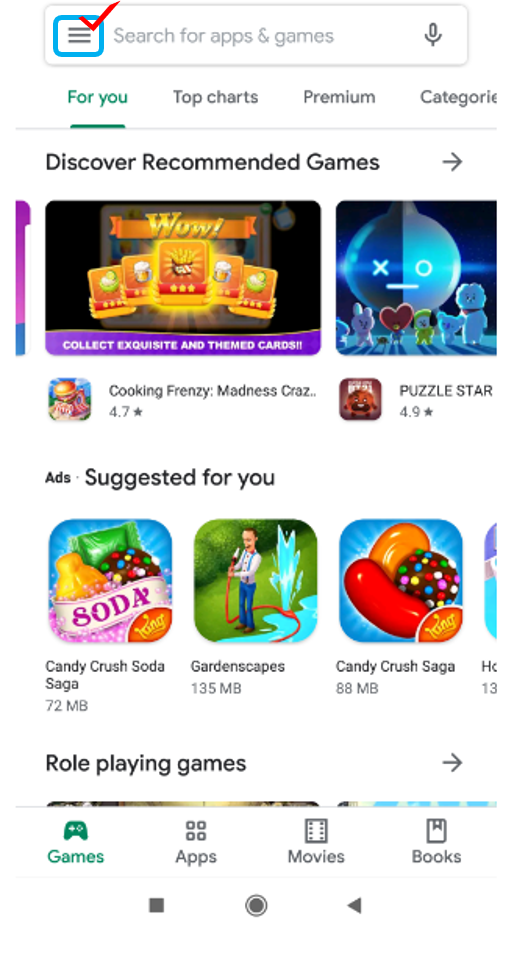The image depicts a mobile app interface predominantly focusing on a gaming and app discovery platform. At the top, there is a search bar accompanied by icons for various functionalities: a hamburger menu with a check mark, and a microphone icon on the far right. Below the search bar, navigation tabs are displayed, including "For You," "Top Charts," "Premium," and "Categories." Among these, "For You" is highlighted in green, indicating it is the currently selected tab, while the others are in gray.

Under the "For You" section, there is a recommendation carousel featuring "Discover Recommended Games" with a right-pointing arrow for further exploration. Noteworthy game suggestions include "Cooking Frenzy Madness Craze," which displays a partially truncated title as "Cooking Frenzy Madness Craz...", with a rating of 4.7 stars. Another highlighted game is "Puzzle Star," boasting a higher rating of 4.9 stars.

The interface also presents "Ads Suggested For You," showcasing games such as "Candy Crush Soda Saga," "Gardenscapes," and "Candy Crush Saga." A separate section for "Role-Playing Games" includes another right-pointing arrow for navigation into more specific game categories.

At the bottom of the interface are additional navigation options for different media categories including Games, Apps, Movies, and Books, each represented by their respective icons: a square, a circle, and a left-pointing triangle.